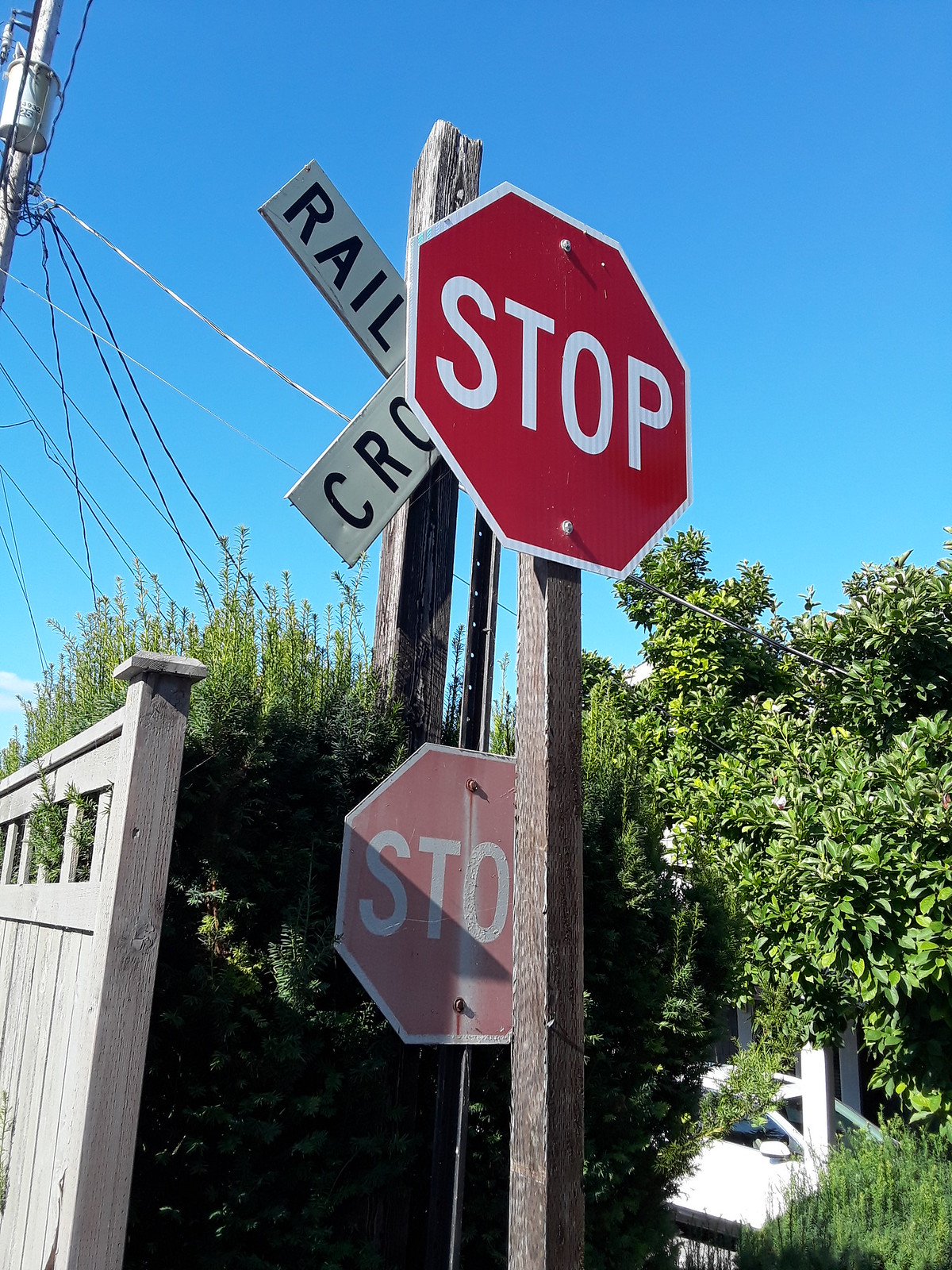This image showcases a detailed and intriguing scene where two stop signs are prominently displayed on dark wooden posts. The first stop sign is positioned higher and is newer, featuring bright red color and crisp white lettering, attached to a square brown post. Below it, the second stop sign appears aged and heavily faded, its red color almost entirely washed out, affixed to a black metal pole. Positioned behind these stop signs is a partially visible railroad crossing sign. The sign reveals only a section of the white diagonal 'X' and the black lettering, with only part of the word "crossing" clearly visible, partially obscured by the higher stop sign.

This arrangement stands against a backdrop of lush greenery with various shades of green leaves and bushes. To the left side of the frame, there is a portion of a light-colored wooden fence, and in the upper left corner, a power box with several wires extends outward. Additionally, the lower right corner of the image shows a section of white fencing. The sky overhead is a clear and bright blue, completing the vivid yet rustic scene.